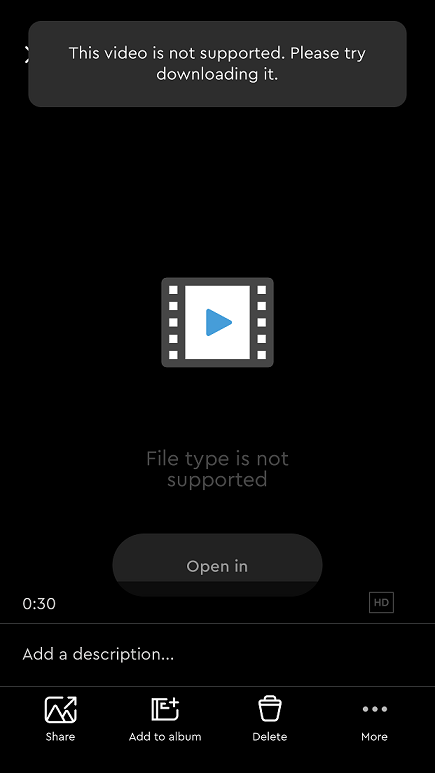The image appears to be a screenshot of a malfunctioning app on a smartphone. The background of the screen is entirely black, creating a stark contrast with the dark gray rectangular pop-up at the top. This pop-up message reads: "This video is not supported, please try downloading it." Below the message is a gray movie reel symbol with a light blue triangle in the center, symbolizing a video file. 

Directly beneath the icon, a second message states: "File type is not supported." Further down, there is a dark gray oval button with the text "Open in" written in white letters. Below this button, the text "30 seconds" appears on the left side of the screen, while "HD" is displayed on the right side. A dividing line separates this information from a text box labeled "Add a description," inviting the user to type in a description.

At the bottom of the screen is a black banner containing several buttons. From left to right, the buttons are labeled "Share," "Add to album," "Delete," and finally, a button with three dots indicating additional options, labeled "More." These buttons are designed to manage the video file, despite the file type not being supported by the app.